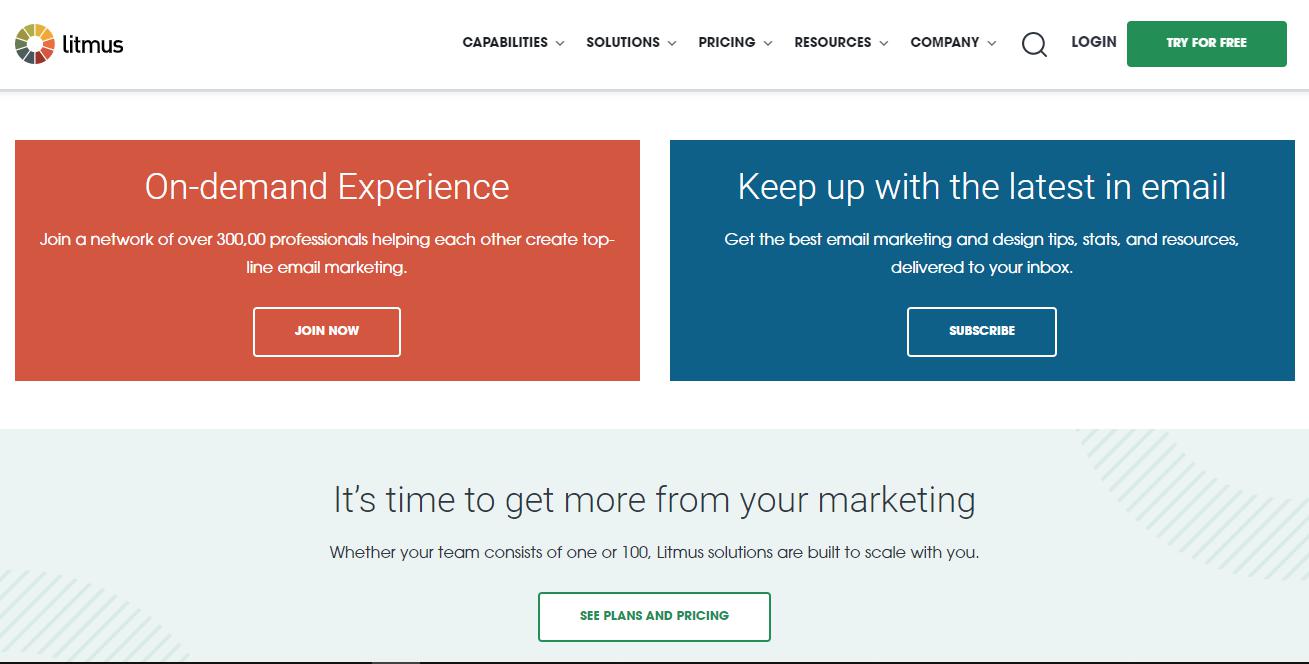In this web page from the company Litmus, the top-left corner features their name and logo. The logo is a multi-colored, thick outer circle with a white inner circle, while "litmus" is written in lowercase black font, all set against a white background. To the right of the logo, there are several pull-down tabs labeled: Capabilities, Solutions, Pricing, Resources, and Company. Additionally, there is a magnifying glass icon for search, a login link, and a green "Try for Free" button with white text.

Below this navigation bar, the page is divided into two rectangular sections. The left section, highlighted in red, has white text promoting an "On-Demand Experience," inviting users to join a network of over 300,000 professionals engaged in top-line email marketing. A "Join Now" link is provided below this message.

The right section emphasizes keeping up with the latest in email marketing. It encourages users to subscribe for the best email marketing and design tips, statistics, and resources delivered directly to their inbox, followed by a "Subscribe" button.

At the bottom of the page, a light blue box stretches across the screen, urging visitors to get more from their marketing efforts. It mentions that Litmus Solutions are scalable, whether for a team of one or one hundred. A "See Plans and Pricing" tab is positioned below this call-to-action.